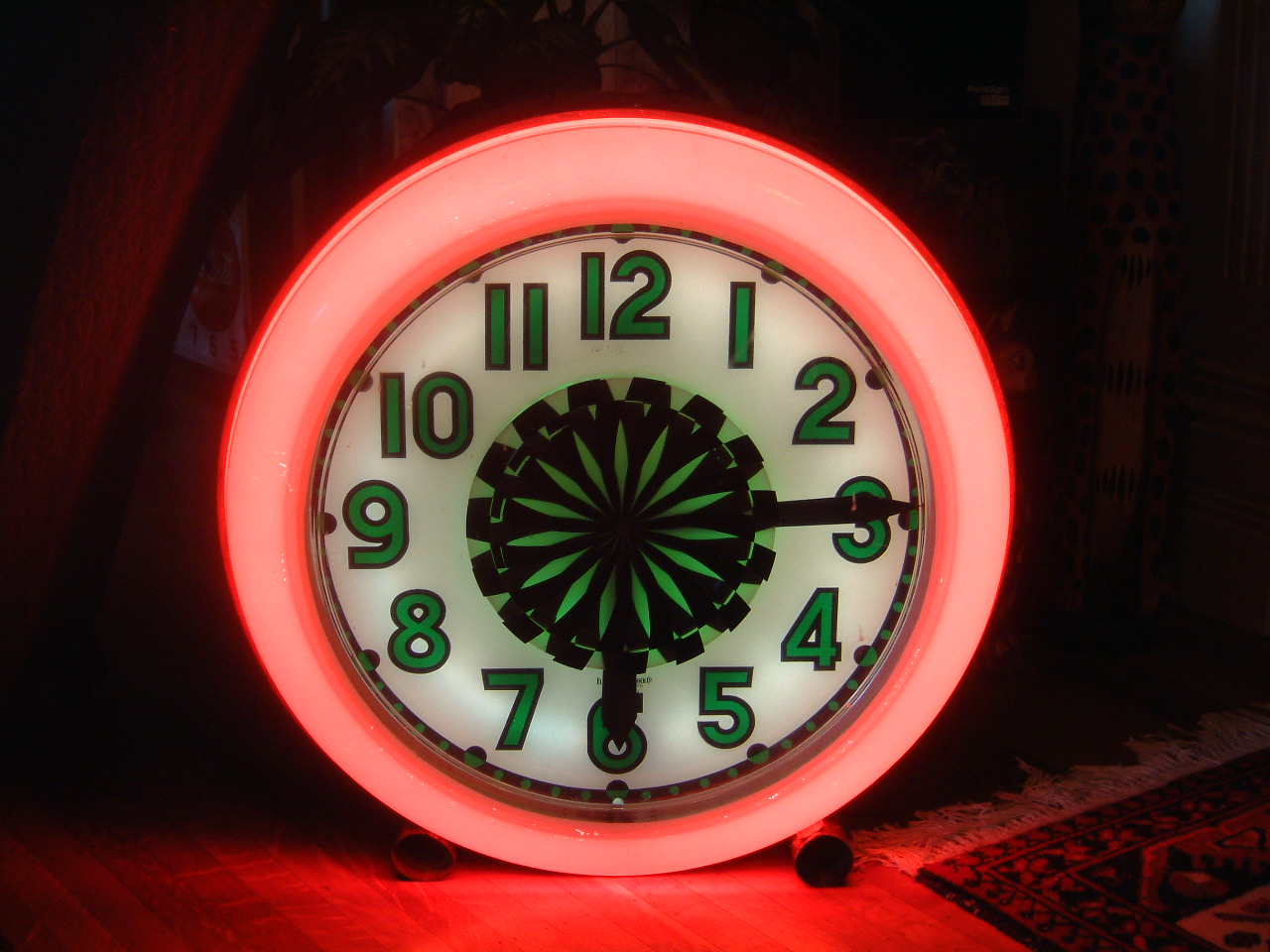This image features a striking and large psychedelic round clock resting on a wooden floor. The clock's design is vivid with a neon red outer ring encircling a white center face. The clock showcases large green numbers, each outlined in black, displaying the time as approximately 14 minutes past 6. The vibrant inner circle radiates with neon green against a black background, resembling a glowing sunburst or a series of interlocking gears, creating an optical illusion of pulsing green and black leaves.

The clock also has two black hands and stands on two round legs, preventing it from rolling. To its right, partially visible, is a detailed rug with white tassels and a pattern of dark blue and red colors. On the left, there is the leg of what appears to be a wooden table. The space behind the clock is not visible in the image.